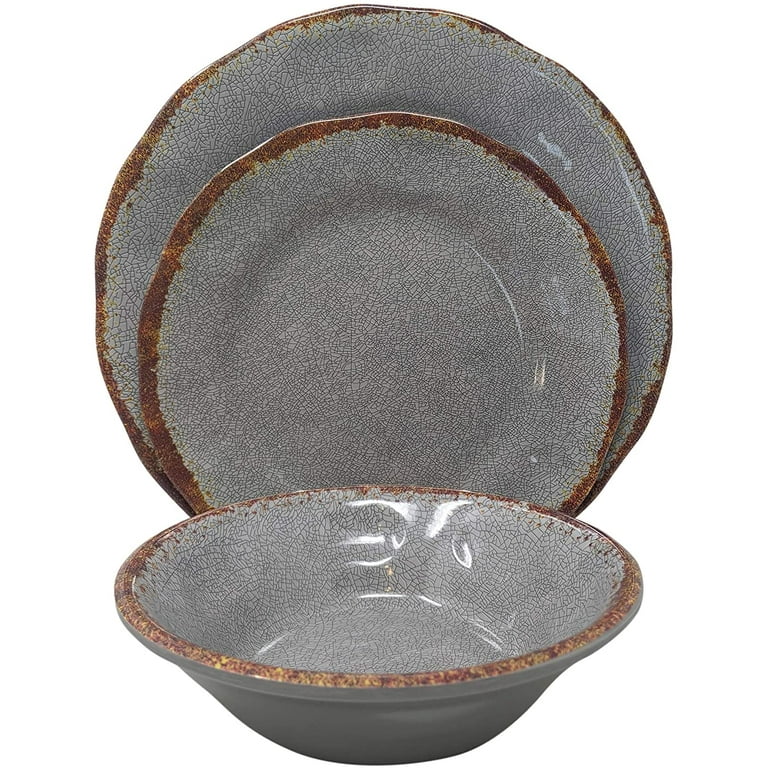The image displays a set of pottery dishes, consisting of a large dinner plate, a smaller salad plate, and a bowl, all arranged against a plain white background. The dinner plate and salad plate are standing upright at the back, with the bowl positioned flat in the foreground. Each piece is characterized by a grayish stone color with a crackling pattern, accented by a bronze or dark rust-colored rim around the edges. The bowl's interior is visible, showcasing its depth and the crackling design. There is a small imperfection, such as a white speck or chip, on the right side of the smaller plate.